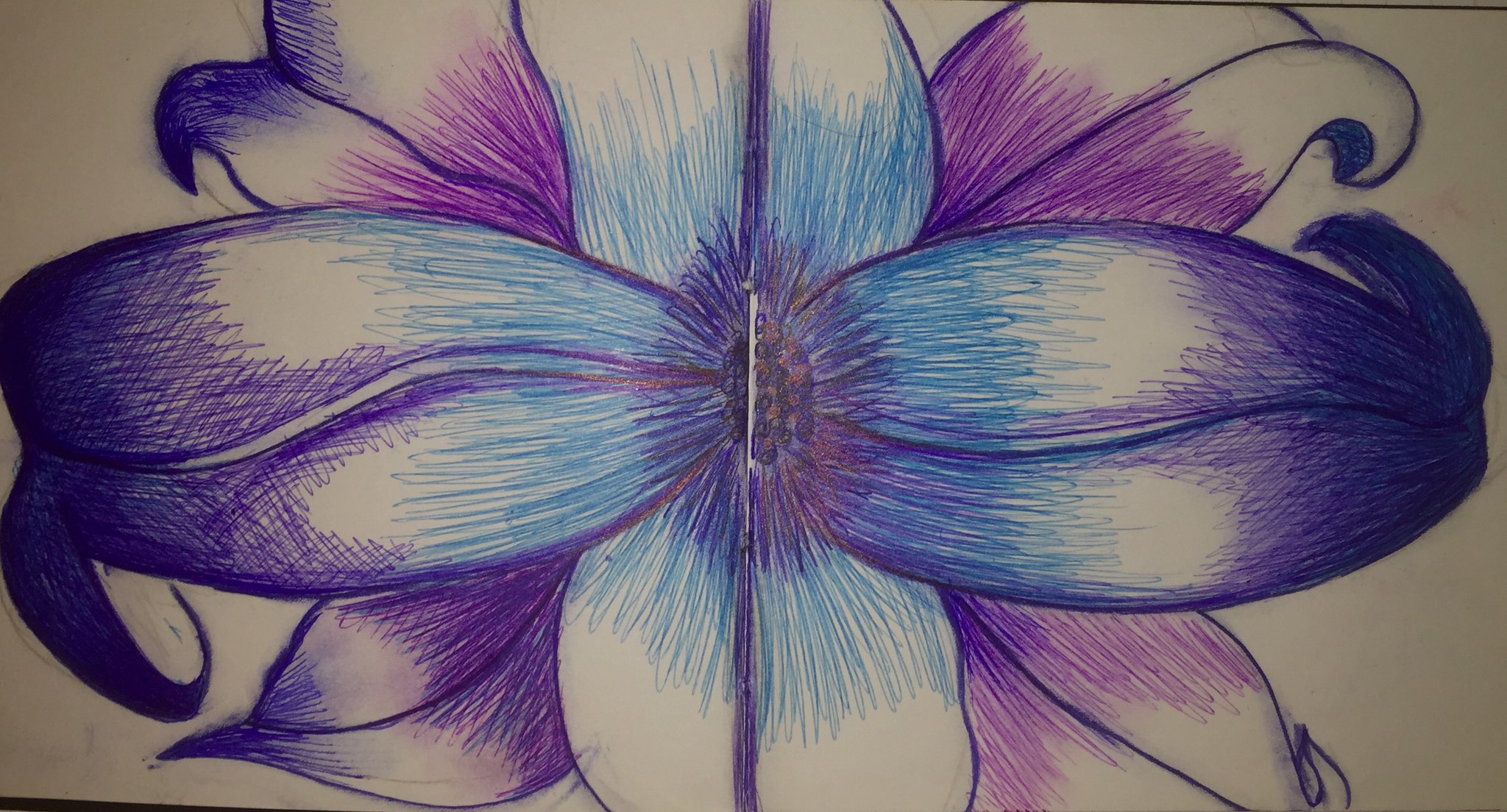This image depicts a detailed drawing of a large, vibrant flower created using ink pens. Displayed on a light brown background, the flower features a total of eight petals. The central part of the flower, thick with stamen-like details, appears in a rich, deep purple, resembling the dense, feathery appearance of eyelashes. The petals radiate outward, colored in meticulously shaded hues. 

Starting with the inner four petals, each begins with blue striations that transition seamlessly into purple towards the tips. The outer four petals mirror this gradient but in reverse; they start with purple at the base, fade into white, and conclude with subtle blue accents at the tips. A dark line runs through the center of each petal, adding to the intricate design.

The flower also demonstrates an artistic play with light, with certain areas left uncolored, imparting a sense of light reflection and depth. The artwork’s use of purple, blue, pink, and white ink pens creates a striking contrast that enhances the flower's vivid and captivating appearance.